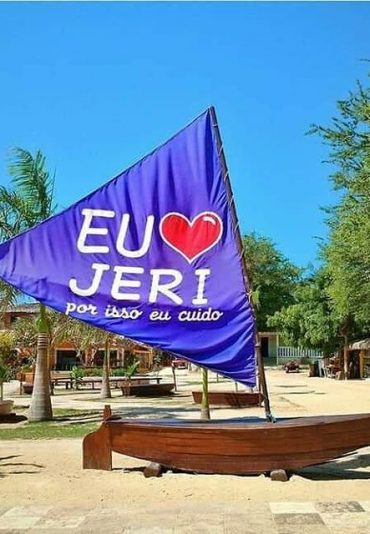The photograph captures an outdoor scene centered around a wooden boat that looks more like a decorative piece than an actual sailboat. The boat, positioned on a sandy or gravel surface with some concrete tiles visible at the bottom, appears to be filled with wood and has a flat top surface. A tall branch serves as a mast for a triangular blue flag featuring large white letters spelling "E-U" with a red heart outlined in white next to it, and "J-E-R-I" below. Underneath "J-E-R-I," in smaller cursive text, are the words "P-O-R-I-S-S-O-E-U-C-U-I-D-O," which seem to be in Portuguese. The boat is situated amidst a backdrop of varied trees—a tall palm tree on the left and larger trees on the right. The top part of the image showcases a clear, vibrant blue sky without any clouds.